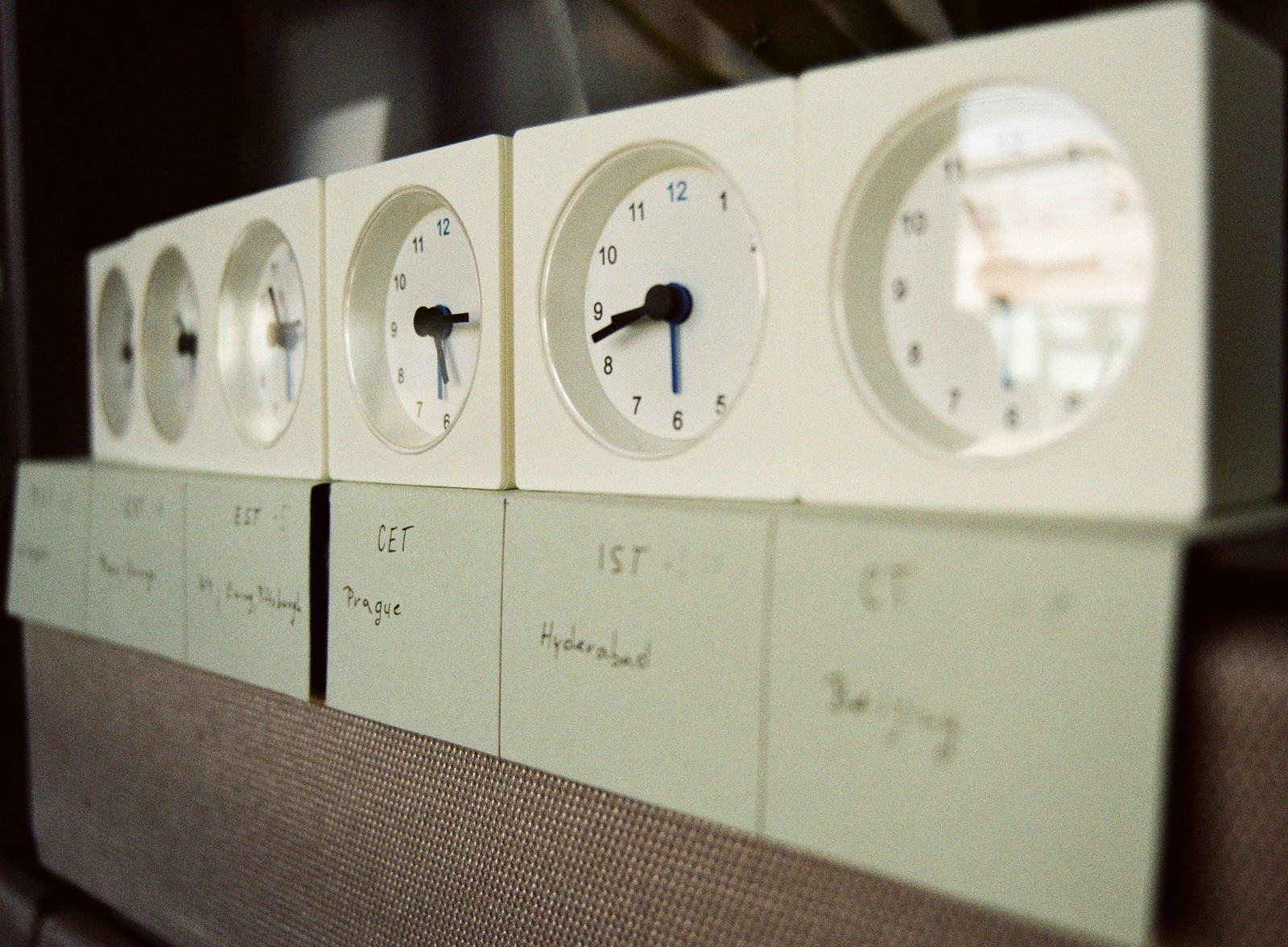The image features six white, cube-like clocks aligned horizontally, each displaying different times, indicative of various global time zones. Each clock has a white face adorned with black numbers; however, the number 12 is highlighted in blue on all clocks. The hour and minute hands are either in a combination of blue, black, or gold and blue, adding a distinct contrast to the minimalist design. These clocks rest on gray blocks that display black text identifying the time zones, though some are challenging to read. From left to right, visible labels read 'First Hyderabad,' 'Get, CET Prague,' and 'CT Beijing,' while the remaining labels are less decipherable. These blocks are positioned on a fabric surface with beige and tan hues, possibly a table or a stand. The backdrop of the image is mostly black, interspersed with some visible poles and a hint of white fabric, possibly a curtain, at the top, framing the setup.